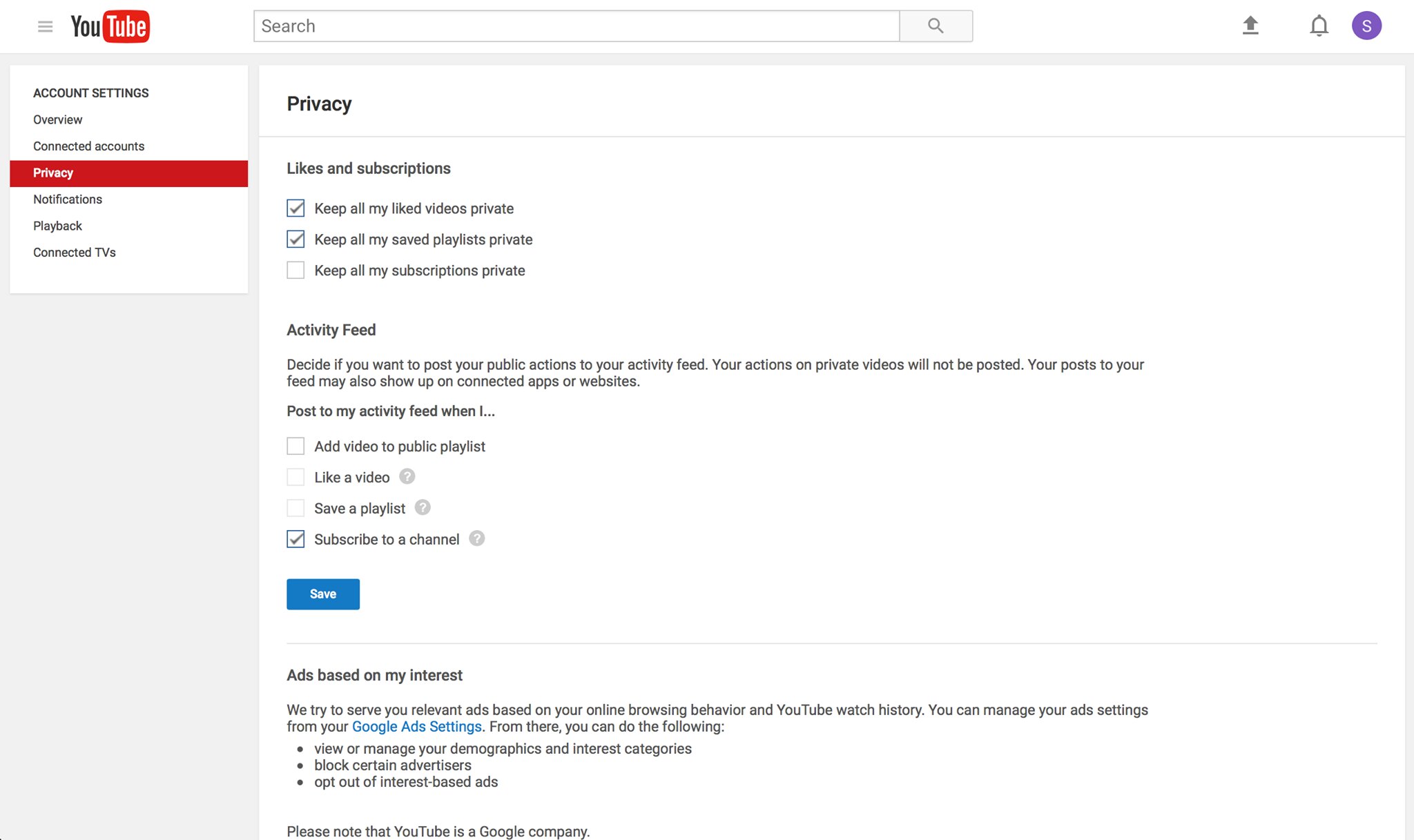The image is a screen capture of the account settings page for a YouTube account. In the top left corner, the YouTube logo and menu bars for navigation are displayed. Below this, a vertical menu lists tabs for Account Settings, Overview, Connected Accounts, Privacy, Notifications, Playback, and Connected TVs. The "Privacy" link is highlighted with a red rectangle, indicating that it is the currently selected section.

Dominating the right-hand side of the screen is the main content area titled "Privacy." Here, several privacy settings are delineated:

1. **Likes and Subscriptions:**
    - The option "Keep all my liked videos private" is checked.
    - The option "Keep all my saved playlists private" is checked.
    - The option "Keep all my subscriptions private" is not checked.

2. **Activity Feed:**
    - A general description explains that users can decide whether to post public actions to their activity feed. Actions involving private videos will not be posted, and these posts may also appear on connected apps or websites.
    - Specific options include:
        - "Post my activity feed when I add a video to a public playlist" (unchecked)
        - "Post my activity feed when I like a video" (unchecked)
        - "Post my activity feed when I save a playlist" (unchecked)
        - "Post my activity feed when I subscribe to a channel" (checked)

3. **Save Button:**
    - A blue rectangular button labeled "Save" is present for saving any changes made to the settings.

4. **Ads Based on My Interests:**
    - A brief explanation states that YouTube attempts to serve relevant ads based on the user's online browsing behavior and YouTube watch history. 
    - Users are informed that they can manage their ad settings via Google Ad Settings, which is a hyperlink.
    - From the Google Ad Settings, users can:
        - View or manage demographics and interest categories.
        - Block certain advertisers.
        - Opt out of interest-based ads.

5. **Disclaimer:**
    - A note at the bottom reminds users that YouTube is a Google company.

At the very top of the image, the URL locator bar, an upload button, a notification bell icon, and a purple circle with the letter "S" in white are also visible.